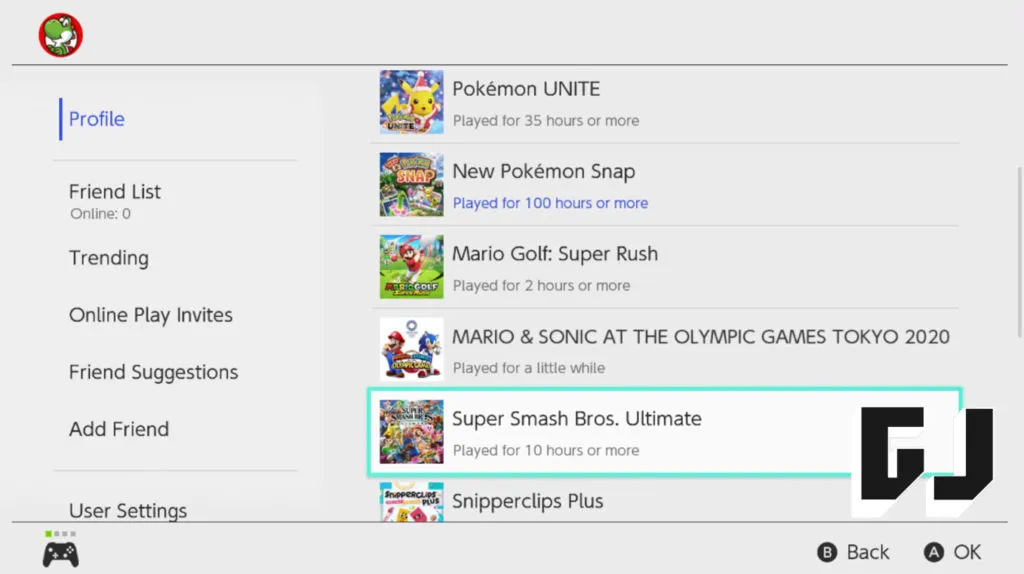This screenshot captures a video game menu in a light gray color scheme. In the top left corner, there is a player icon featuring Yoshi against a red background, indicating it is Player 1 with a video game controller icon situated in the bottom left. On the bottom right, the menu provides two options: the "B" button labeled "Back" and the "A" button labeled "OK."

Dominating the screen is the menu itself. On the left side, there's a vertical list of options: "Profile," "Friend List," which further lists "Online Zero," "Trending," "Online Play Invites," "Friend Suggestions," "Add Friends," and "User Settings." To the right of this, there is another list of game options. At the top is "Pokemon Unite," followed by "New Pokemon Snap," "Mario Golf: Super Rush," "Mario and Sonic at the Olympic Games Tokyo 2020," "Super Smash Bros. Ultimate," which is highlighted with a selection rectangle, and finally "Snipperclips Plus."

In the bottom right corner, a large icon displays the stylized letters "GJ," adding a distinct visual element to the interface.